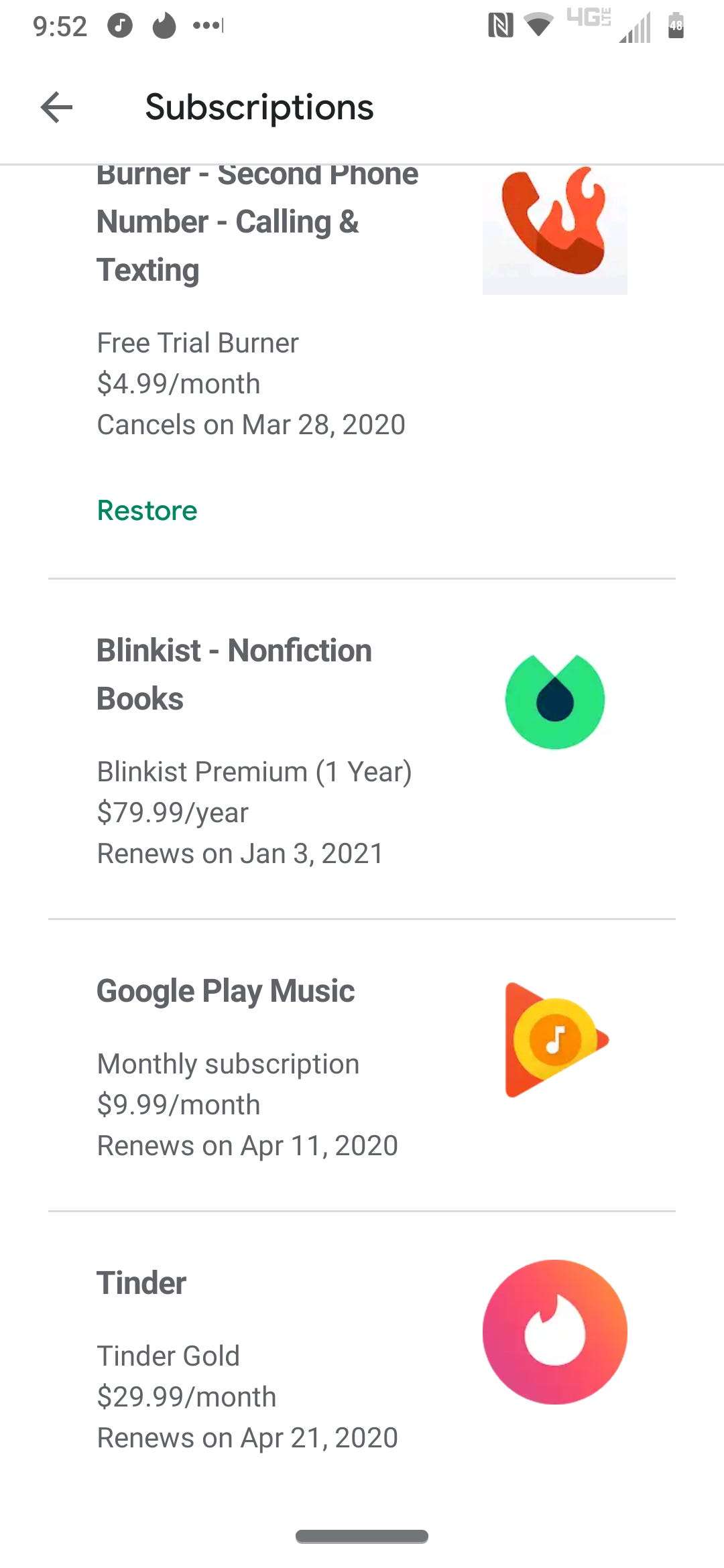A detailed snapshot taken from the Google Play Store app, showcasing the "Subscriptions" page. The background is white with black font, and at the top, the title "Subscriptions" is prominently displayed. The body of the snapshot features four distinct subscriptions:

1. **Burner: Second Phone Number, Calling, and Texting**  
   - **Description:** Free trial for Burner  
   - **Cost:** $4.99 per month  
   - **Status:** Cancels on March 28, 2020

2. **Blinkist: Nonfiction Books**  
   - **Description:** Blinkist Premium, one year  
   - **Cost:** $79.99 per year  
   - **Status:** Renews on January 3, 2021
  
3. **Google Play Music**  
   - **Description:** Monthly subscription  
   - **Cost:** $9.99 per month  
   - **Status:** Renews on April 11, 2020
  
4. **Tinder**  
   - **Description:** Tinder Gold  
   - **Cost:** $29.99 per month  
   - **Status:** Renews on April 21, 2020